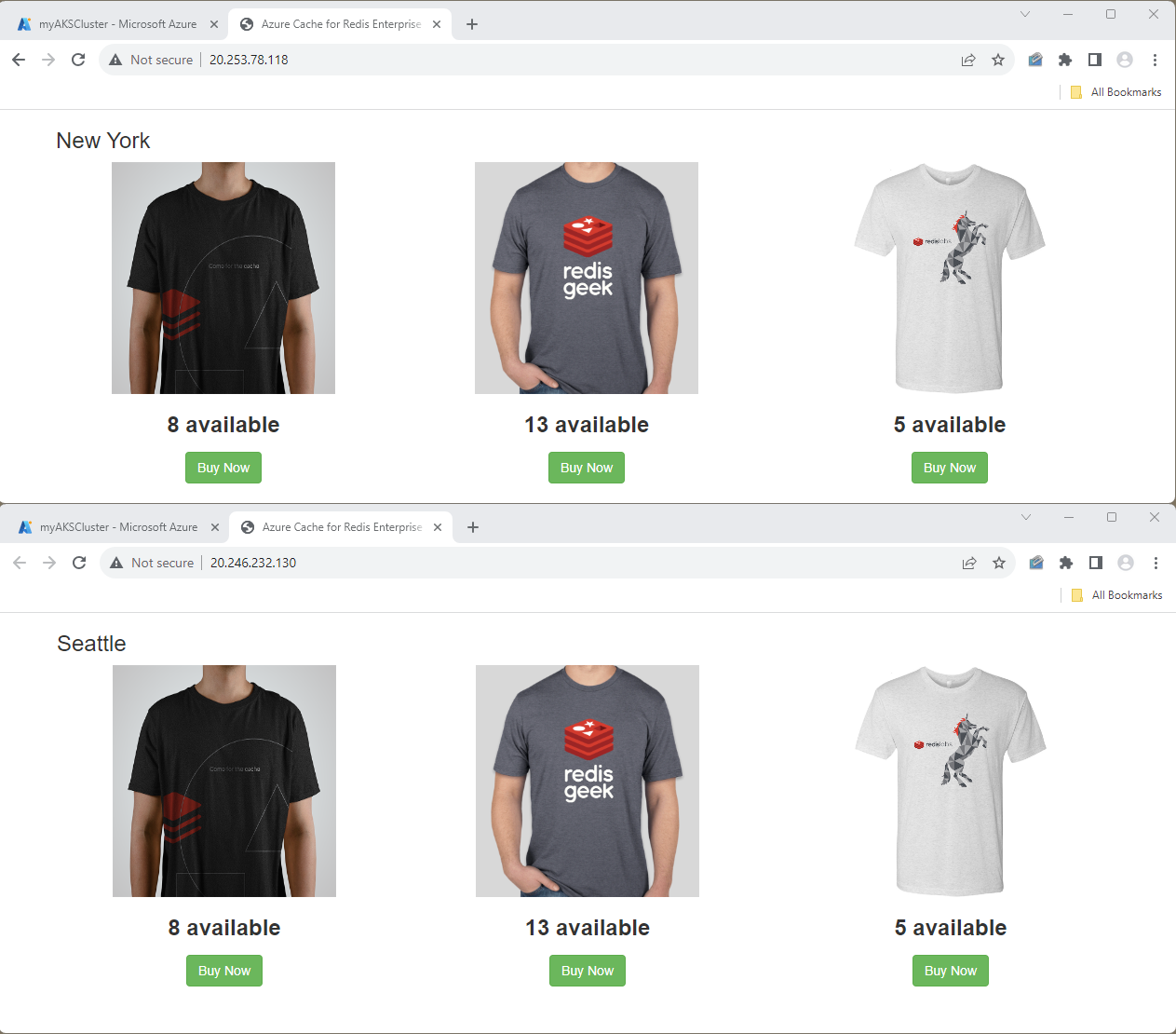The image displays a split view of a website interface showcasing Microsoft Azure services and an e-commerce section.

The top section features a light gray banner with the text "my AKS Cluster" (with "AKS Cluster" in capitalized letters as one word) and "Microsoft Azure." An active tab reads "Azure Cache for Redis Enterprise." This section has a white background and icons for navigation: a left arrow, a right arrow, and a refresh button, with the left arrow and refresh icons in darker colors. The address bar shows a warning sign (a triangle with an exclamation mark) indicating "Not Secure," followed by the IP address "20.253.78.118." Below the address bar, the content switches to a white background displaying "New York."

Under the "New York" section, a series of t-shirts are listed:
1. A t-shirt labeled “8 available” in a green box, accompanied by a white "Buy Now" text.
2. Another t-shirt with “13 available,” also in a green box with "Buy Now" in white.
3. A standalone white t-shirt with “5 available” in a green box and "Buy Now" in white.

The bottom section mirrors this setup but indicates a different IP address, "20.246.232.130," and location "Seattle." The availability and "Buy Now" options for the t-shirts align with the New York section.

Overall, the image provides a detailed view of the Azure dashboard alongside an e-commerce platform offering various t-shirts, differentiating between New York and Seattle locations.